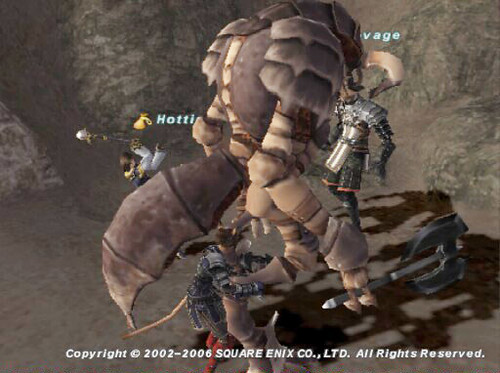A screenshot from an early 2000s 2D game, boasting primitive yet charmingly vintage 3D graphics, shows an intense battle scene. Three human characters engage in combat against a formidable, armored beetle wielding a double-sided axe in its right hand and sporting a large, steel-armored stinger tail. One character attacks its legs beneath the armored tail, another confronts it from the front, and a third stands behind the tail, waving a staff. The scene, rendered in grainy, pixelated visuals, captures the nostalgic essence of early gaming. At the bottom of the image, the caption "© 2002 to 2006 Square Enix Co., Ltd. All rights reserved." suggests that this retro game was developed by the renowned company Square Enix.